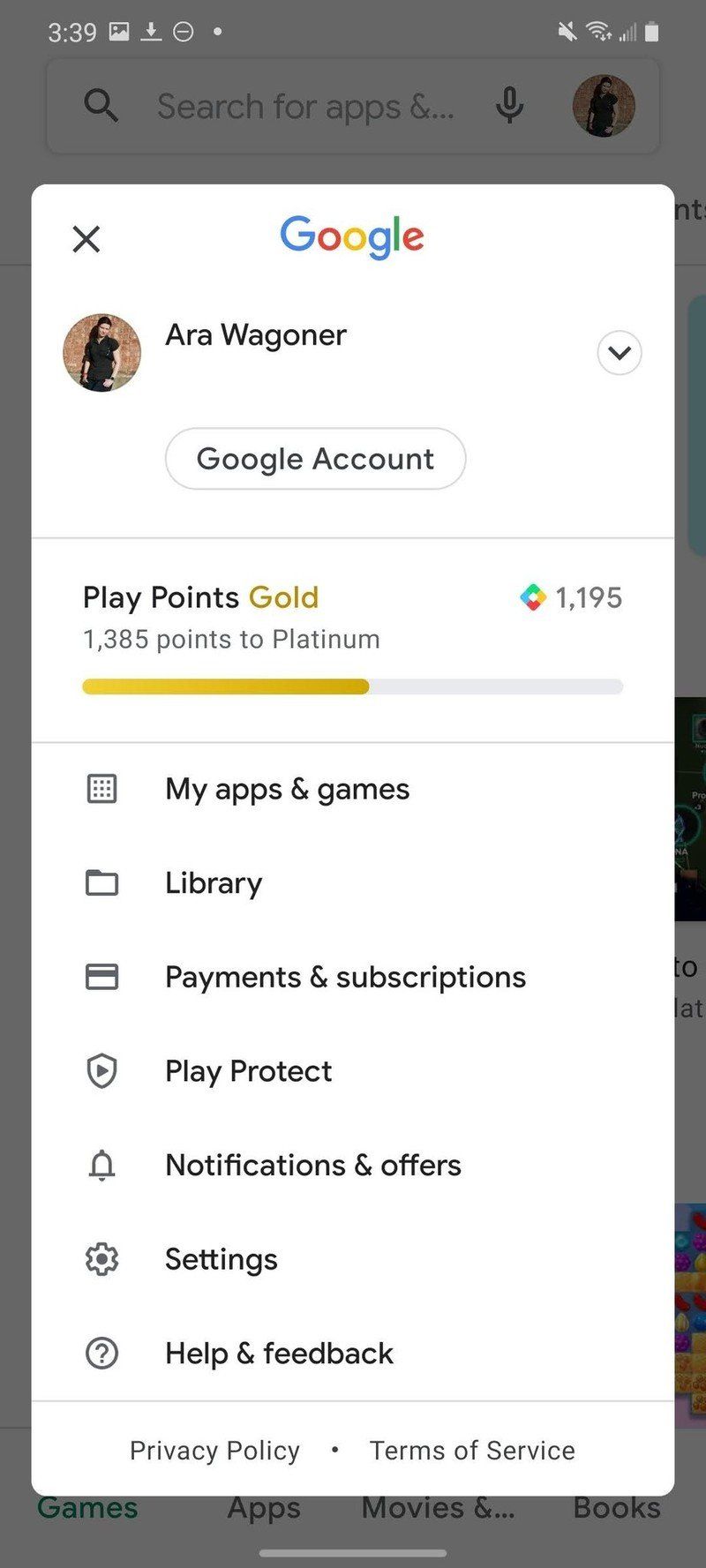The image appears to be a screenshot from the Google Play Store app, displayed against a gray background. In the top left-hand corner, there is the number "339" along with three icons: a photo icon, a download arrow icon, and a no access icon. The upper right-hand corner shows several status indicators including no sound, Wi-Fi, data signal, and battery life icons.

At the forefront of the image, there's a white text box with a black 'X' in its upper left corner designed to close the box. Below the 'X', the Google logo is displayed in its signature blue, red, yellow, and green colors. A profile image of a person wearing a black shirt and pants is visible, identified as "Aria Wagner Google account."

Within the same box, details regarding Play Points are shown: Aria has accumulated 1,195 points and needs 1,385 points to reach platinum status, with a half-filled gold bar illustrating this progress. The menu below this includes categories such as "My Apps and Games," "Library," "Payment and Subscriptions," "Play Protect," "Notifications and Offers," "Settings," "Help and Feedback," "Privacy Policy," and "Terms of Service."